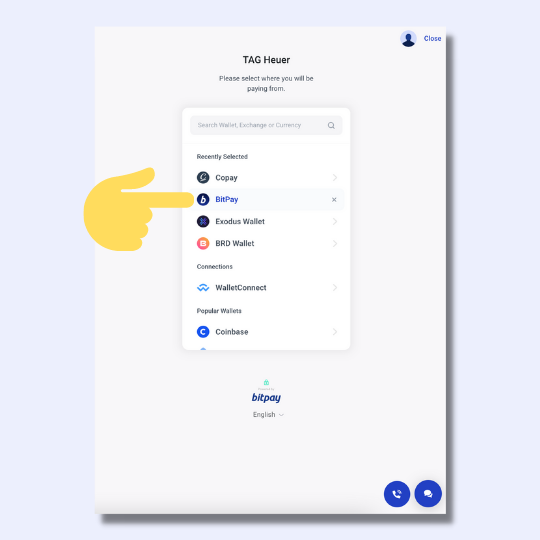The image features a screenshot with a light grayish purple background. At the center of the screenshot is a prominent white rectangle. In the upper right corner of this rectangle, there is an icon representing a person next to the word "Close."

In the center of the screen, bold black text reads "Tag here. Recently select where you will be paying from." Below this text is another white box with a search bar at the top, labeled "Recently Selected." Within this box, several payment options are listed:

1. **Copay**
2. **Bitpay** (highlighted in blue, with an illustrated hand pointing to it)
3. **Exodus Wallet**
4. **BRD Wallet** (displayed as an orange 'B' in a circle)

Further down, there is a section titled "Connections" which features an icon resembling a wave of water next to the text "Wallets Connect."

Below this, the "Popular Wallets" section includes:
- A white 'C' inside a blue circle labeled "Coinbase"
- The Bitpay logo, also in blue

This detailed layout outlines the various elements and options visible in the screenshot, providing a clear and comprehensive description of the image’s content.